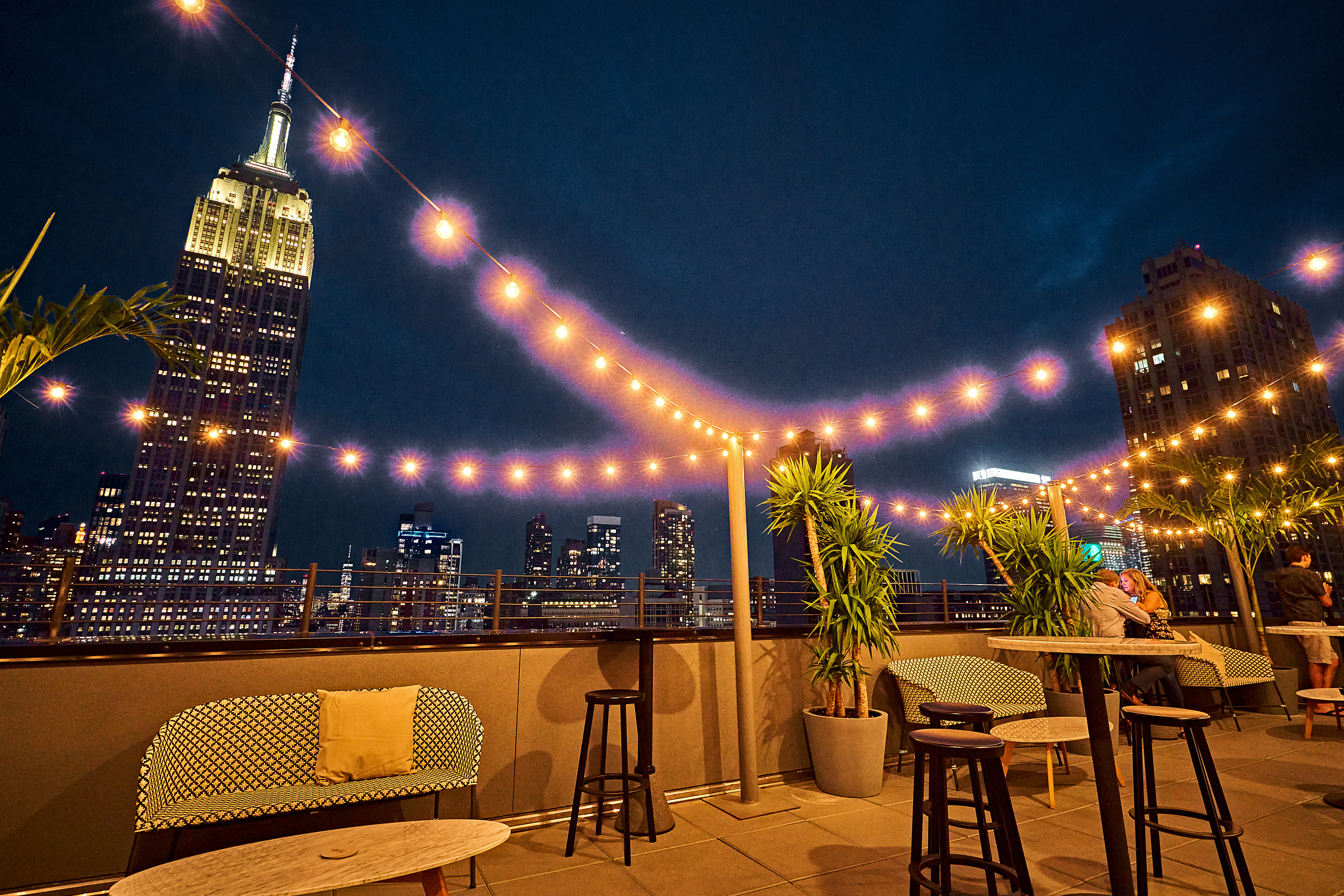The nighttime rooftop scene captures a cozy, bustling ambiance on a rectangular photograph measuring approximately 5 to 6 inches wide and 4 inches high. The picture showcases a rooftop deck of a building, providing a stunning view over a city skyline adorned with illuminated skyscrapers in the background. The wall of the roof, a light brown color, can be seen starting in the lower left-hand corner, ascending about an inch before extending towards the right-hand side. Below, the floor is laid with brown tiles, creating a warm, inviting surface for the rooftop furniture.

The rooftop is furnished with an eclectic mix of amenities, including tall bar tables with stools and lower couches made from thin, weather-resistant materials. These couches are accompanied by uniquely shaped coffee tables resembling surfboards or ovals. Potted plants, some tropical in nature, occupy various spots on the deck, adding a touch of greenery. Additionally, several tall clay pots house short trees.

Adding to the charm of the scene, strands of little bulbs cross in X-shaped patterns overhead, emitting light that is white in the center and transitions to a pink or purplish-pink hue on the outside. The deep blue night sky provides a serene backdrop for these lights, enhancing the overall atmosphere. The rooftop is alive with activity; some people are seated at tables conversing, while others stand, capturing the vibrant surroundings with their cameras. This detailed photograph encapsulates a perfect blend of urban elegance and lively social interaction.